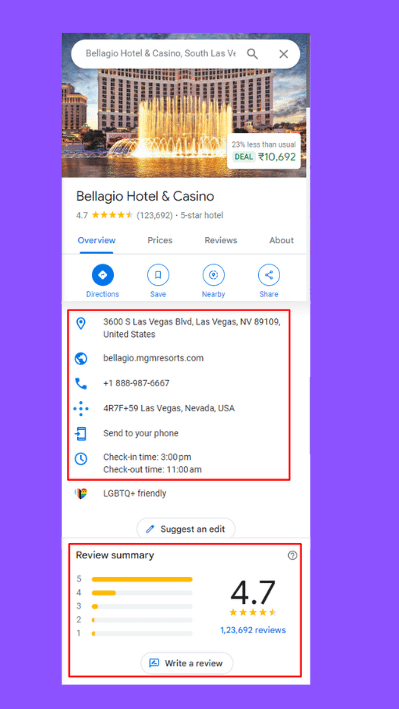![Bellagio Hotel and Casino Website Interface](image-link)

The screenshot depicts the official website interface of the Bellagio Hotel and Casino, located in South Las Vegas. The search bar at the top shows the user has looked up this renowned establishment. Dominating the main visual is an impressive picture of the Bellagio, a distinguished curved white building. The image captures the enchanting moment of sunset, with the sky blending into dusk hues while the bottom portion remains illuminated. Adjacent to the Bellagio on the left is another standing structure.

In front of the Bellagio lies an enormous fountain set within a pond, adding to the aesthetic appeal. A small box near the pond indicates a promotional deal, stating "23% less than usual," accompanied by the number "10,692," which likely isn’t in American currency. 

A prominent banner displays that the Bellagio Hotel and Casino has achieved a rating of 4.7 stars out of 123,692 reviews, emphasizing its five-star status. The webpage offers navigational tabs such as "Overview," "Prices," "Reviews," and "About," with "Overview" highlighted in blue, indicating it's the current selection.

Below these tabs, users can find icons for "Directions," "Save," "Nearby," and "Share." Information within a red-outlined white box includes the hotel's address, website, phone number, additional address, options to send details to a phone, and check-in and check-out times (3 p.m. and 11 a.m. respectively), each accompanied by blue icons.

A multi-colored heart icon signifies the hotel's LGBTQ+ friendly status, accompanied by the text in gray. Further down the page, another white box with a gray outline invites users to "Suggest an edit."

The review summary section, framed in a red-outlined white box, prominently displays a 4.7-star rating based on 123,692 reviews, with detailed statistics shown in blue. This section visualizes feedback distribution with bars for each star rating, predominantly filled for five stars. Users are encouraged to write a review, with the option highlighted in black at the bottom, accompanied by a blue-outlined white box for submission.

Overall, the interface provides a comprehensive overview of the Bellagio Hotel and Casino, emphasizing its luxurious offerings and high customer satisfaction.